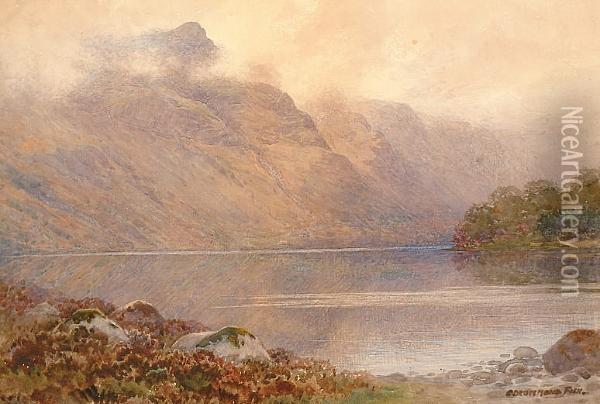This landscape painting, possibly an oil or watercolor piece, depicts a serene scene of a lake surrounded by mountains. The image features a rocky and green shoreline in the foreground, with short vegetation and a mix of small and large stones, as well as pine cones and leaves scattered about. The calm, rippled lake reflects the towering brown mountains in the distance, their tops shrouded in dense fog or clouds. The mountains stretch across the entire backdrop, giving a sense of vastness, while the muted, washed-out colors of the mountains contrast with the vibrant greens and browns of the foreground. White clouds float above, glowing with a hint of orange or yellow, adding warmth to the painting. On the right-hand side of the shoreline stands a cluster of green trees, while an island with taller trees can be seen in the center of the lake. The bottom right corner of the painting has a small, almost illegible artist's signature, and “niceartgallery.com” is written vertically along the right-hand side. The overall composition conveys a light-colored, tranquil atmosphere.